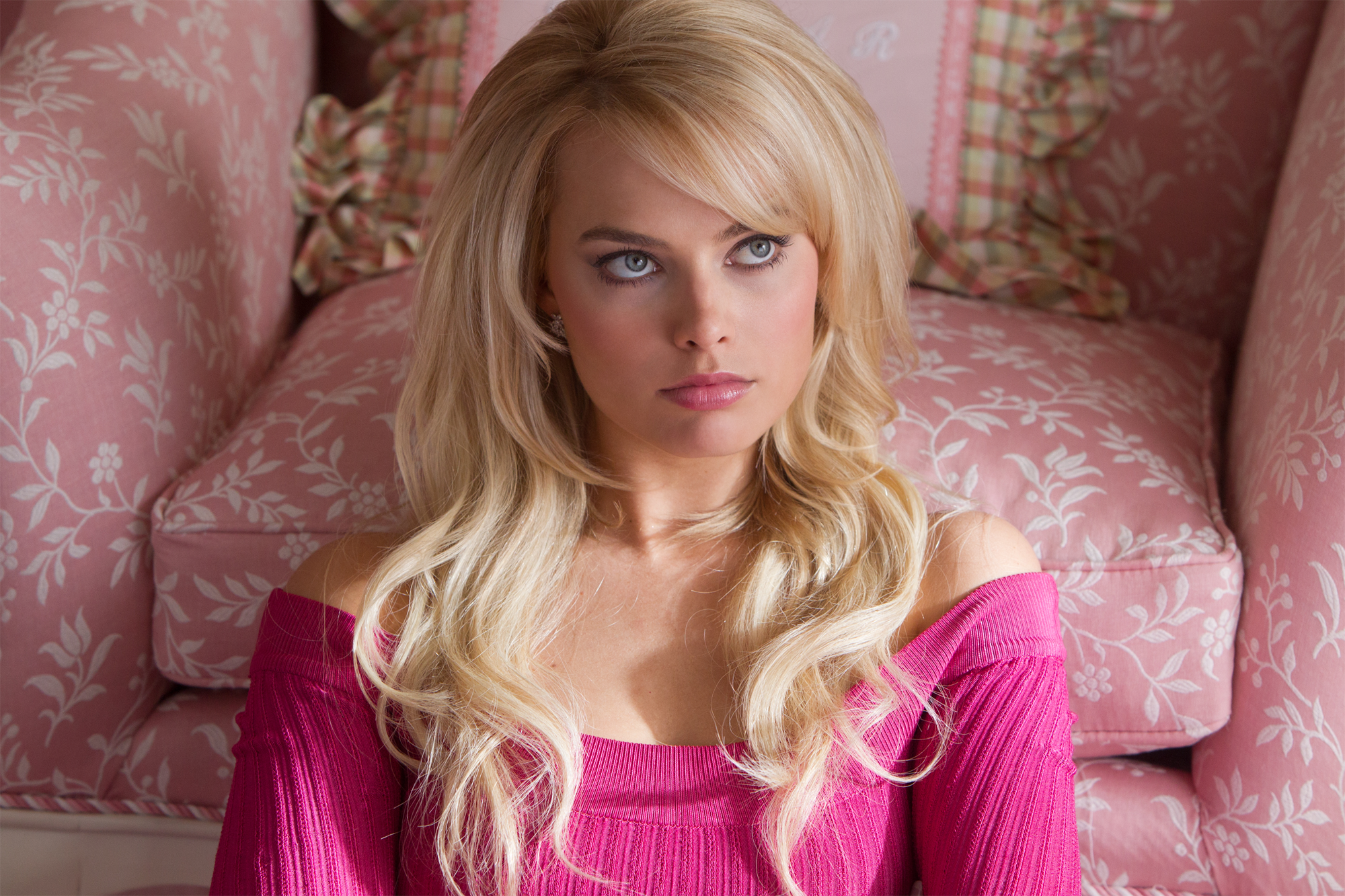In this detailed movie still, a woman resembling actress Margot Robbie is seated on the ground in front of a plush, peach-pink chair adorned with intricate white floral embroidery. Her long, wavy blonde hair cascades over her shoulders, complementing her pink, off-the-shoulder ribbed sweater that exposes her collarbones. This exquisite chair features a pink, green, and white plaid throw pillow with ruffled edges and a central pink square, adding a touch of whimsy. The delicate braided trim along the chair’s bottom edge enhances its softness and elegance, while the woman’s slightly displeased expression brings an interesting depth to the image.